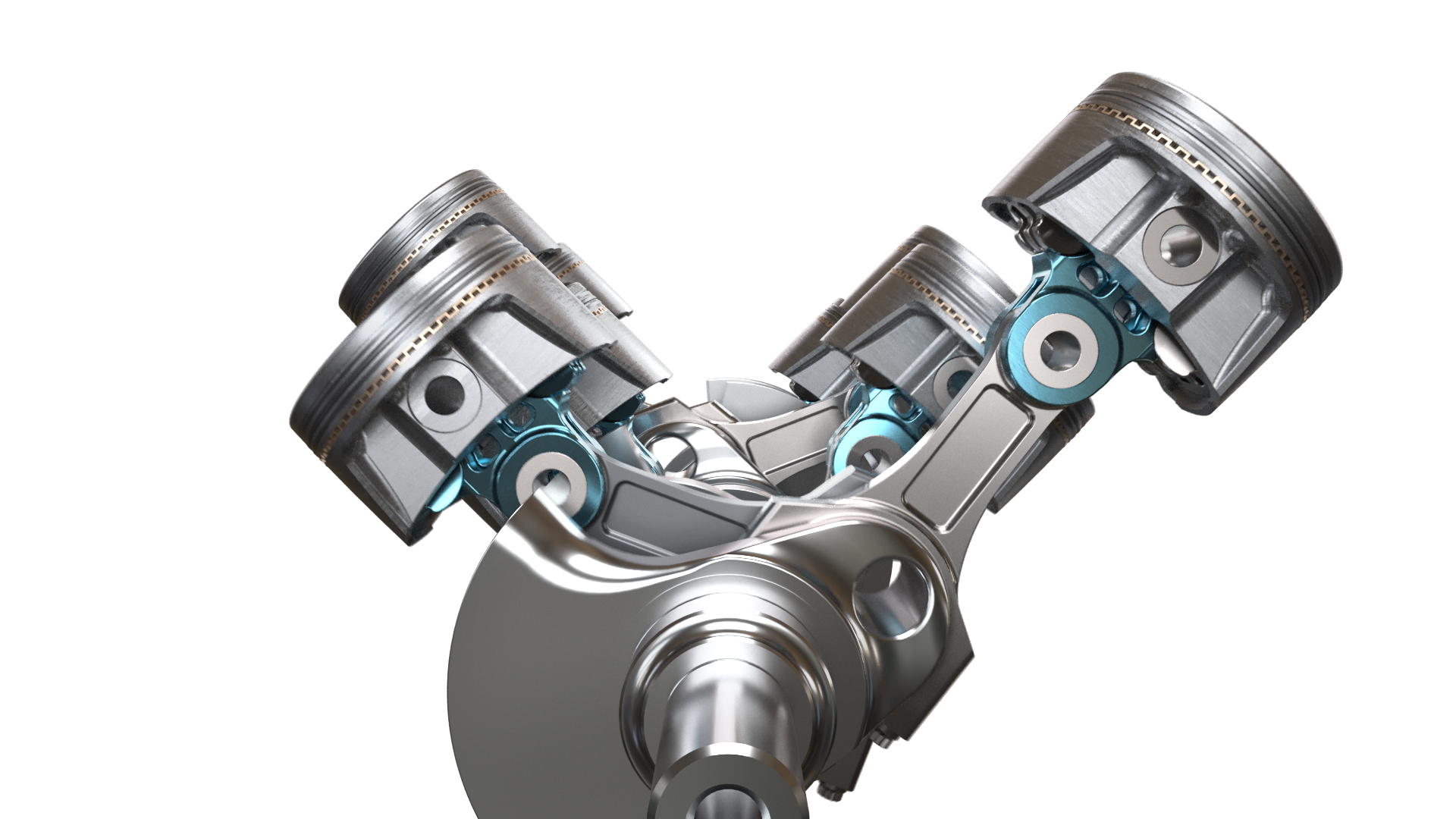This digital illustration features a highly detailed, silver-toned mechanical component set against an entirely white background. Central to the image is a cylindrical structure extending outward, leading back into multiple interconnected parts. The primary body comprises a rod-like apparatus adorned with four piston-like cylinders, positioned in a V formation—two in front and two more staggered behind. Each piston is capped in silver and features a distinctive gold line just below the cap. The pistons are secured with bolts that are encircled by a light blue ring followed by a white ring. Additionally, small red box-like markings can be found on the tops of the pistons. The precise details and the high-definition nature of the illustration accentuate the metallic, industrial aesthetic of the component, suggesting advanced engineering akin to automotive technology.